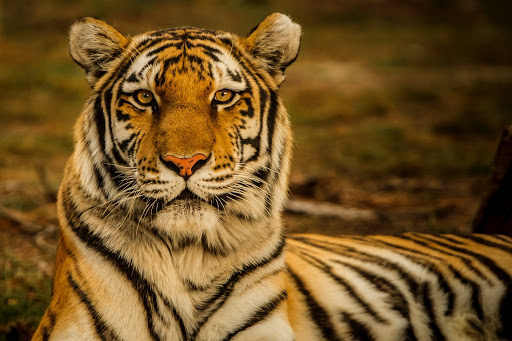This close-up photograph features a tiger looking directly into the camera, giving it an alert and confident demeanor. The majority of the image captures the tiger's head and neck, showcasing its distinctive orange fur with white and black stripes. The nose, a prominent feature, is slightly more reddish-orange compared to the rest of its fur. White whiskers fan out from the snout, and the tiger's orange-green eyes stand out vividly. The background, a blurred brownish-green, suggests the photo was taken during daytime and highlights the focus on the tiger's striking gaze and majestic appearance. Its ears appear slightly dusty, enhancing the raw and natural feel of the image. The photograph excludes the tiger's legs, emphasizing its powerful head, upper body, and the top of its back.